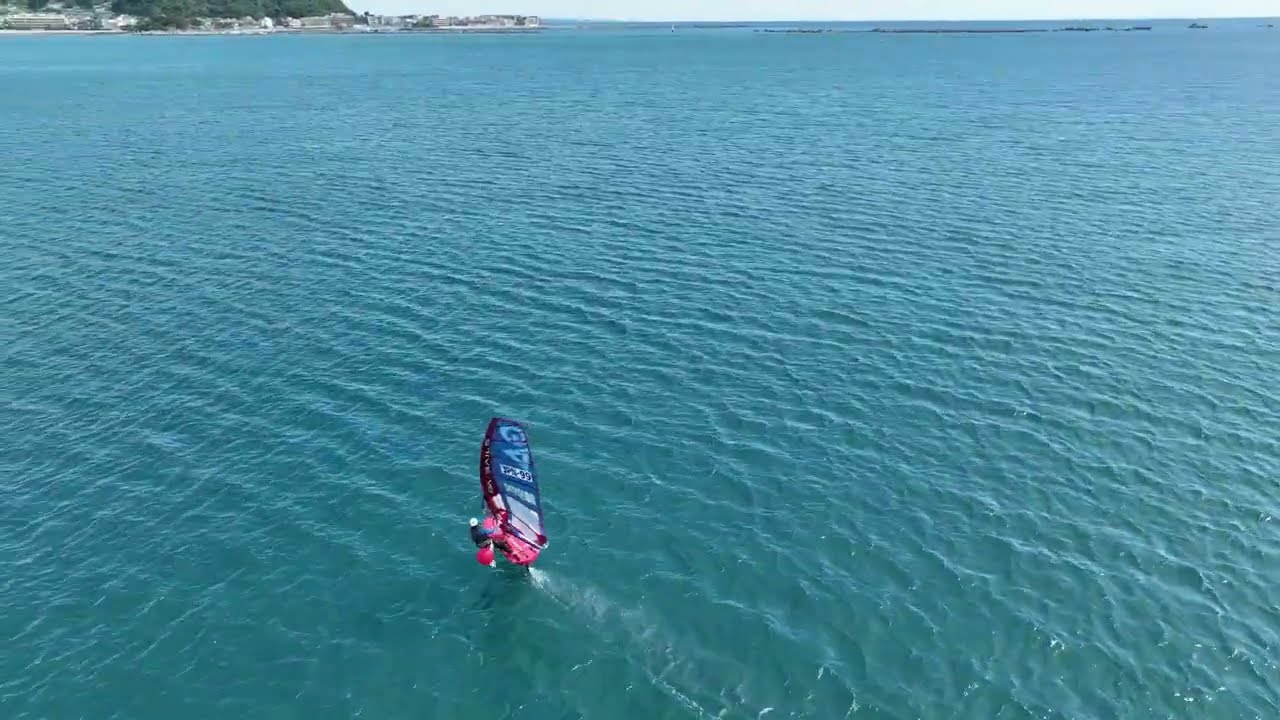The photograph captures a vibrant outdoor water scene dominated by the turquoise blue expanse of the sea or ocean. Stretching across most of the image, the clear, slightly wavy waters exude a tropical allure. In the foreground, a person stands on a small red-bottomed watercraft that features a distinct sail, primarily black and blue with some white lettering. This sail suggests either a parasailing setup or a unique wind-powered craft, seemingly almost suspended above the water. The person, donned in a blue shirt and possibly a pinkish lower garment, wears a white item on their head. In the background, the upper left corner reveals a distant shoreline with visible buildings and greenery, along with a mountainous area marked by patches of white, possibly cliffs, indicating a rocky terrain. The land and its structures add depth to the serene yet dynamic maritime landscape, drawing the eye towards the horizon where the sea meets the sky.